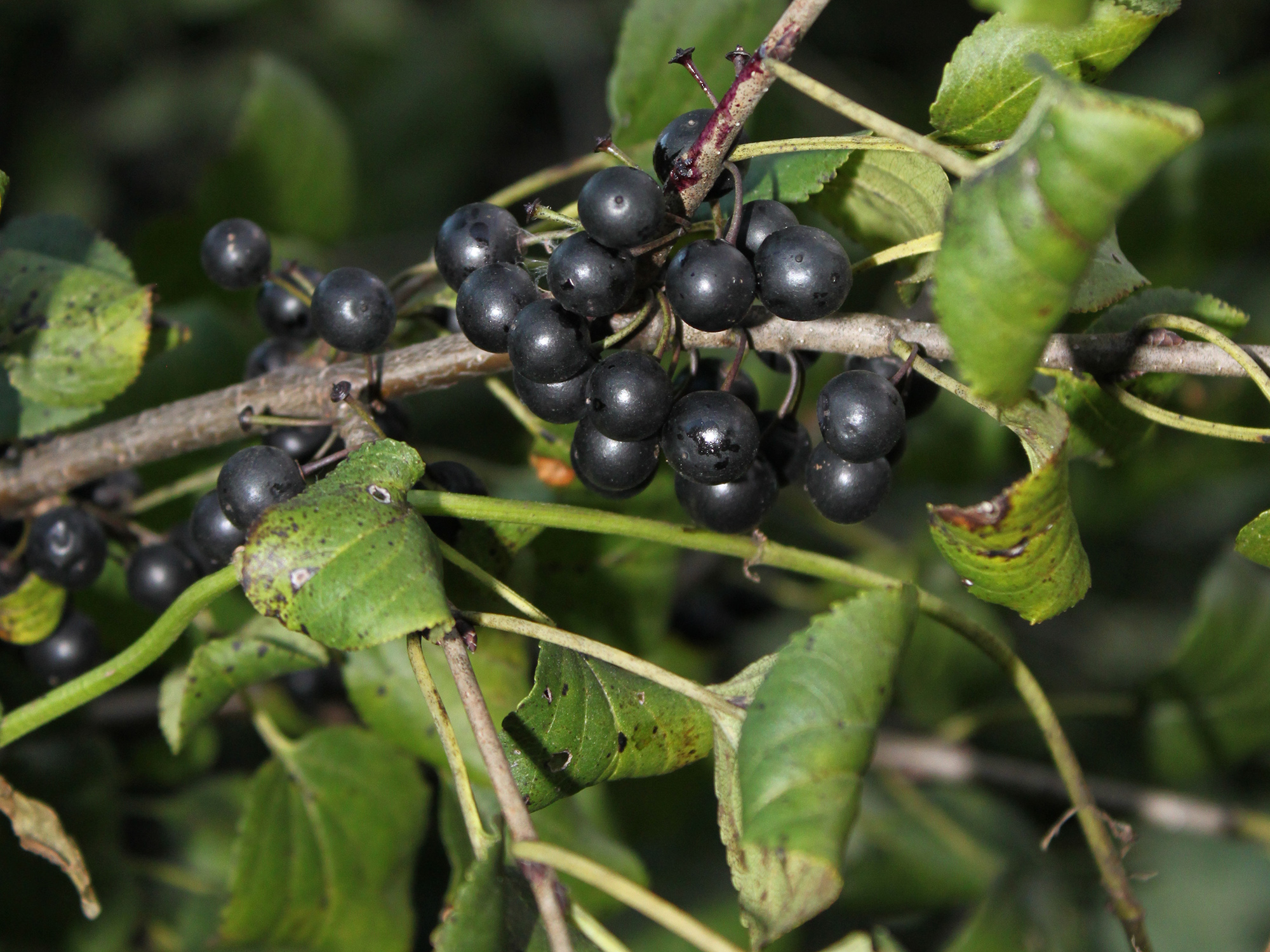A highly detailed and close-up shot captures a cluster of approximately 15 circular, bluish to dark blue berries growing centrally on a brownish stick. Surrounding this primary cluster are additional smaller clusters of berries positioned towards the bottom left of the stick, though these are less prominent. The berries, which have an almost navy hue, are set against a backdrop of green leaves, some of which curl inward, adding texture to the image. The background is intentionally blurred, hinting at more leaves and sticks in darker tones, which further emphasizes the sharpness and vividness of the main subject. The scene suggests a natural abundance, with leaves sprouting in varied shades of green and yellow, some appearing on lighter stems. The careful composition highlights not only the berries but also the intricate details of the leaves and stems, enhancing the organic aesthetic of the photograph.